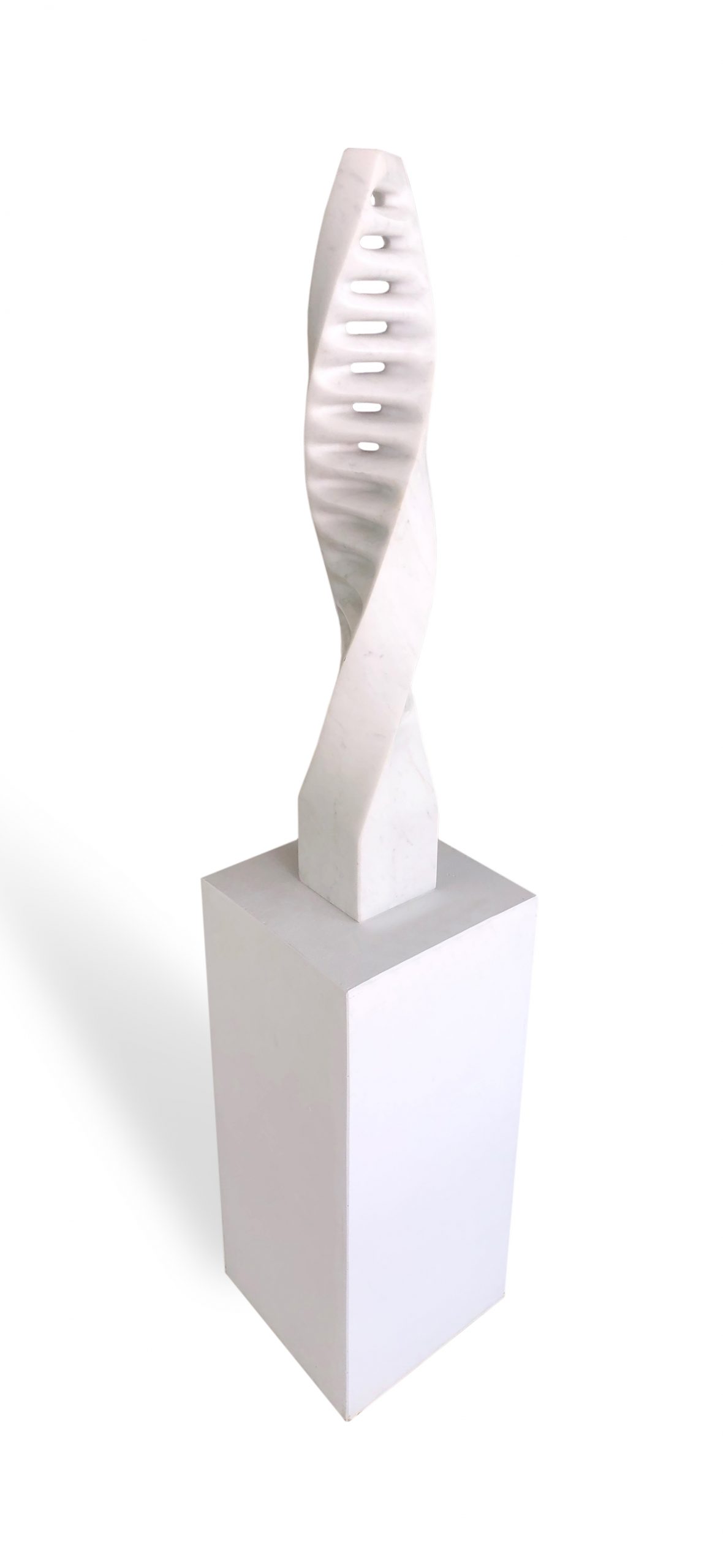This photograph depicts a modern sculpture with a minimalist, clinical aesthetic. The sculpture stands against a completely white background, emphasizing its stark and precise geometry. The base is a tall, elongated, rectangular pedestal made of whitish-gray marble. Positioned atop the pedestal is a striking double helix structure, reminiscent of a DNA strand, crafted from the same marble material. This DNA-like spiral features two parallel strands joined by symmetrically spaced interconnecting bands, creating an intricate pattern of open negative spaces. The entire piece is bathed in subtle shadows, highlighting the variations in shading between the different elements. The spiral, which is approximately the same height as the pedestal, narrows slightly towards the top, enhancing the dynamic sense of twisting motion.